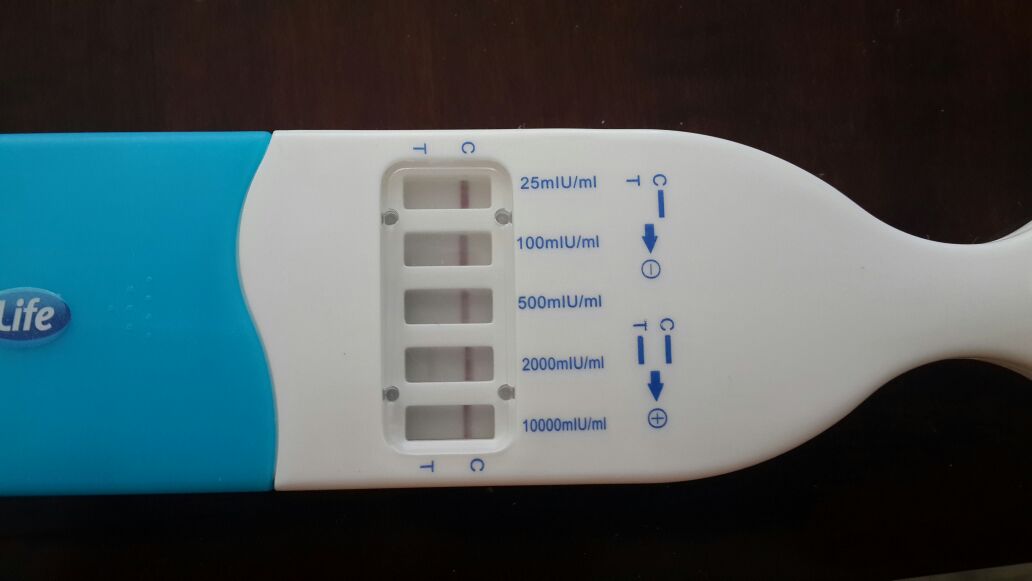In this close-up color photograph, a pregnancy test is prominently displayed on a wooden table, with the grain of the wood serving as the background. The test is taken at an angle that highlights the device in detail. The upper part of the test stick is white, marked with blue text that shows a guide: the letters "C" and "T" indicating the control and test lines, respectively. The guide also explains that one line signifies a negative result, while two lines indicate a positive result. The lower part of the stick is blue, featuring the word "Life" in a white font inside a blue circle. The test window, centrally located, shows noticeable control and test lines, along with measurement increments including 25, 100, 500, and 1000 milliliters. The photograph clearly illustrates these features, providing a comprehensive view of the pregnancy test device and its markings.